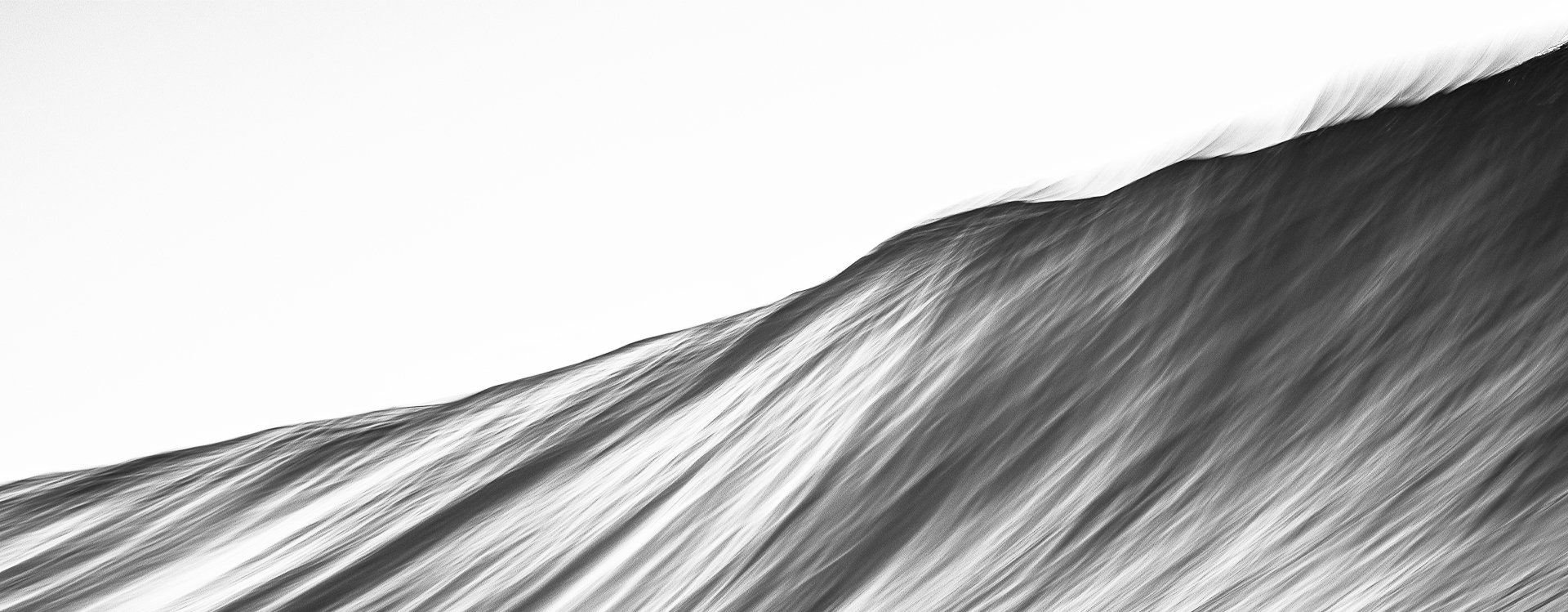This rectangular black and white piece of art predominantly features an intricate illustration of a wave. The image is much longer horizontally than vertically, creating a dynamic scene that extends across the canvas. The wave starts from the bottom left corner and rises diagonally to the top right, with its crest just beginning to curl over on the upper right side. The top portion of the artwork is mainly white, gradually blending into gray towards the upper left-hand corner. This white area at the crest resembles the foamy peak of a breaking wave. The shading throughout the piece utilizes various tones of black, gray, and white, giving it a textured, almost pencil-drawn quality. The tapered arrangement of colors from the bottom to the crest enhances the illusion of a powerful, rising wave, with the thicker white and gray areas on the left side emphasizing the wave's form and movement.